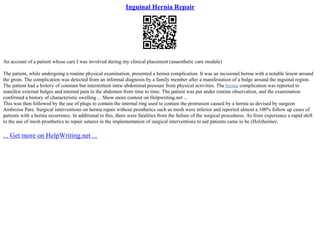This blurry, small rectangular image features a title in a medium royal blue font at the top, reading "Inguinal Hernia Repair," the first word being underlined. Below this title is a QR code. Further down, there are approximately ten lines of very small, left-justified black text, with the first line separated by a space from the subsequent lines. The text is largely unreadable except for the word "the" beginning the first paragraph. In the bottom left corner, also left-justified, is blue text in the same shade as the title, though not bold, stating, "...get more on helpwriting.net..."